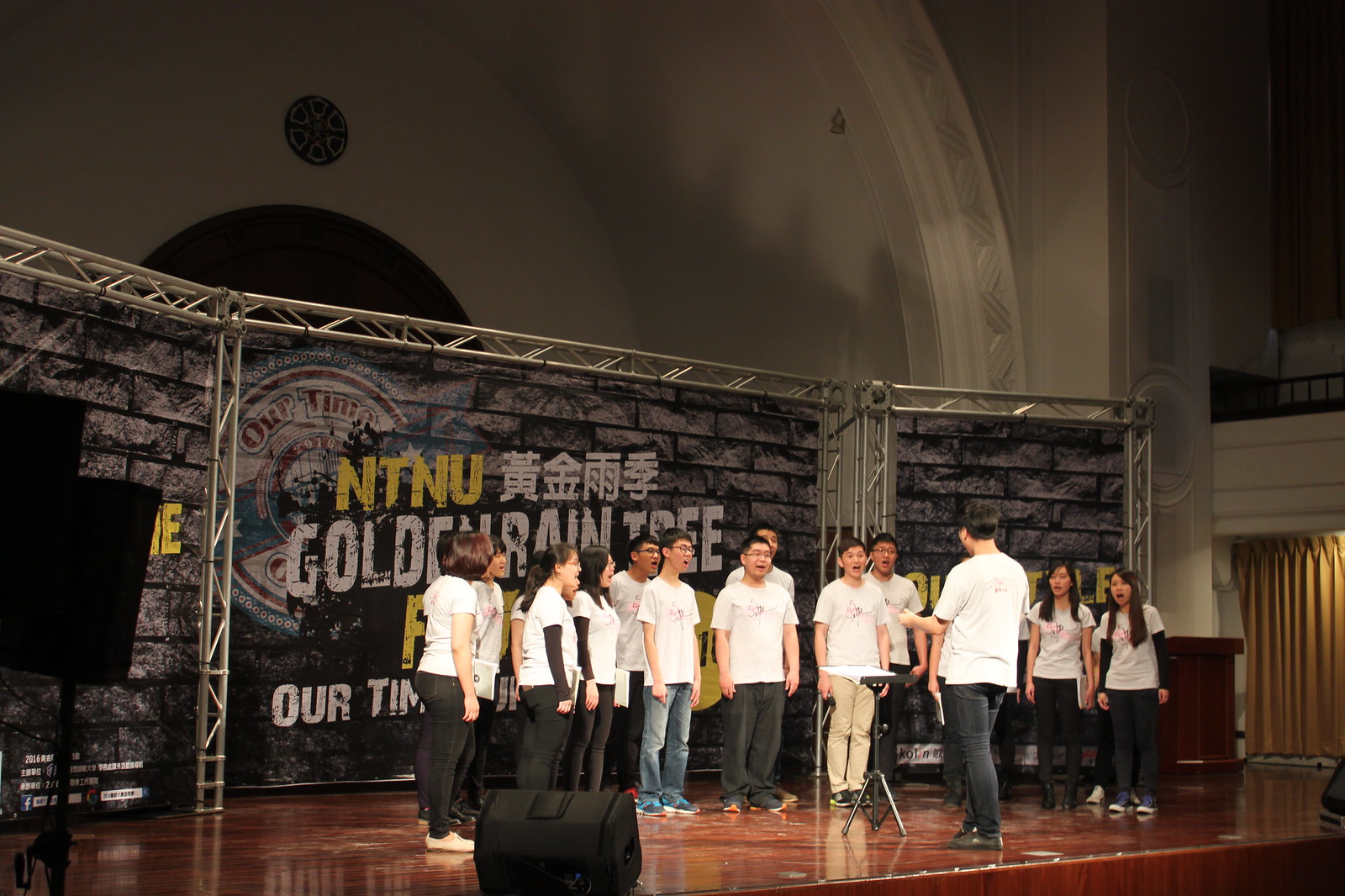The image depicts an indoor concert or recital featuring a group of Asian students, likely teenagers, standing on a stage with a shiny brown floor and red curtains. They are all dressed in white shirts and black pants, with few wearing blue jeans or khaki pants. These students appear to be singing, their mouths open and eyes forward, possibly engaged in a choral performance or competition. 

In front of them stands an Asian man in a white short-sleeved shirt and black pants, facing away from the camera and seemingly conducting the choir. His arms are raised, and a music stand with sheet music is positioned before him.

Prominently displayed behind the choir are large banners designed to look like brick walls. The central banner reads "NTNU" in gold letters, followed by Asian characters and the English words "Golden Rain Tree." Similar banners are on either side with partially visible words ending in "E." Above the banners, the top of the image features an arched wall painted in a light color, possibly white or light gray, giving a semblance of an ornate music hall. The overall atmosphere suggests a formal yet earnest event, dedicated to showcasing the musical talents of these young singers.